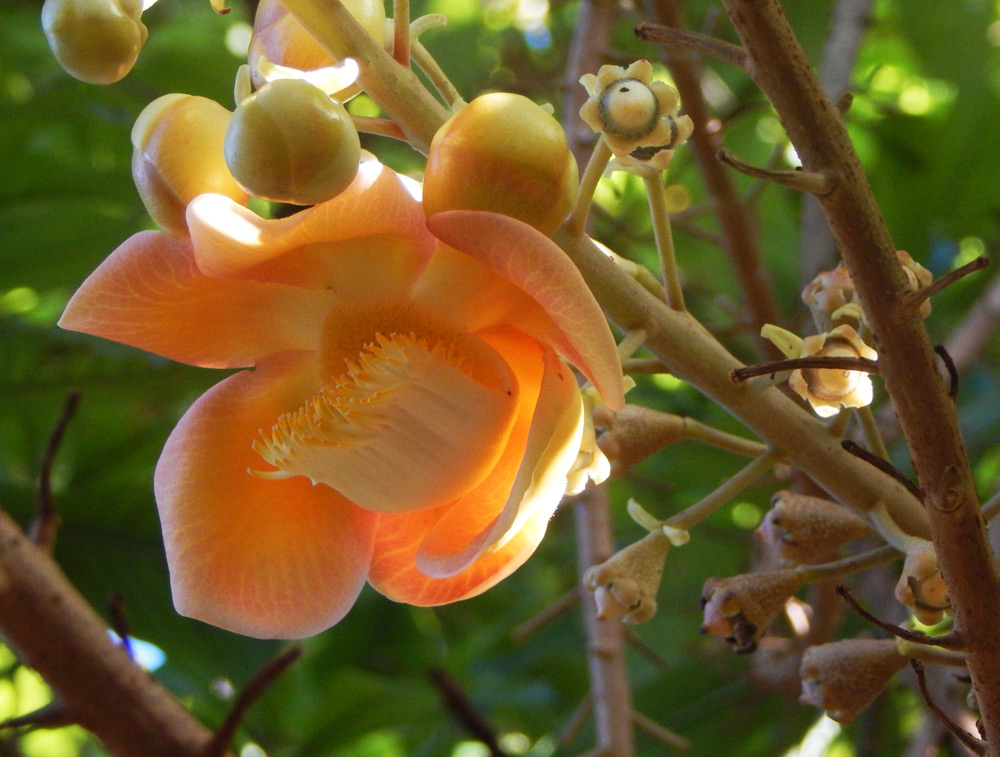The image captures a detailed macro shot of a robust, peachish-orange flower, nearly fully bloomed, flaunting its sturdy, thick petals that appear almost rubbery. The center of the flower reveals prominent pistils that are wispy at the ends. Surrounding the flower, large yellow acorns, some unripened, cling to the tree's branches, with blooming and budding stems rich in yellowish-orange hues. Out of focus in the background, the green leaves of the tree weave together, occasionally letting small glimpses of blue sky and sunlight peek through, casting subtle shadows and adding depth to the scene.